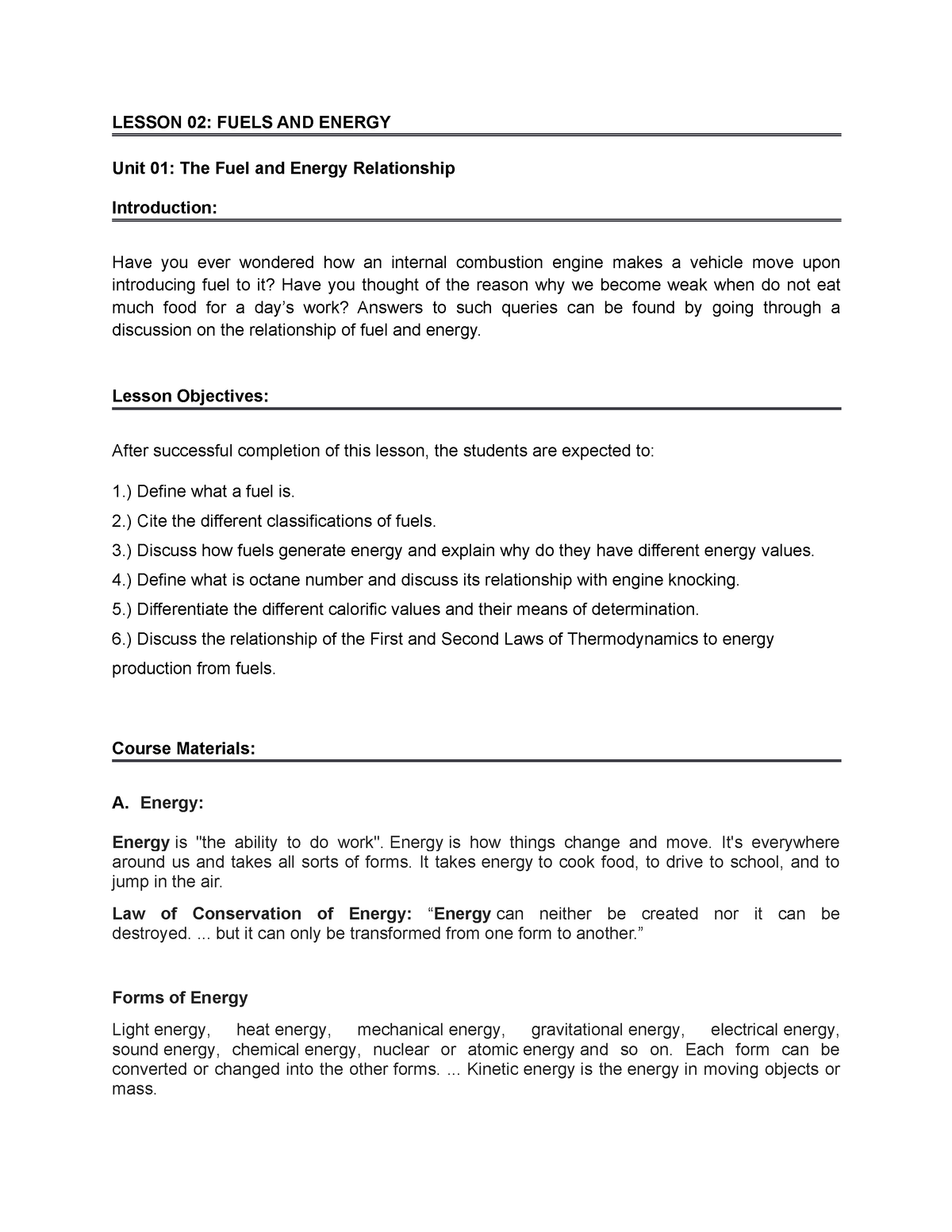In the image, the background is white, providing a clean and uncluttered visual context for the content. The central feature is a blueprint-style heading that states "Lesson 02: Fuels and Energy." Below this, a blue line serves as a separator, followed by the text "Unit 1: The Fuel and Energy Relationship."

The lesson begins with an "Introduction" section, marked by another line. This section prompts students with engaging questions: "Have you ever wondered how an internal combustion engine makes a vehicle move upon introducing fuel to it?" and "Have you thought about why we become weak when we do not eat enough food for a day's work?" These questions serve as a gateway to understanding the intricate relationship between fuel and energy.

Following the introduction, the "Lesson Objectives" are outlined, emphasizing the key learning outcomes for students. By the end of the lesson, students should be able to:

1. Define what fuel is.
2. Cite the different classifications of fuels.
3. Discuss how fuels generate energy.
4. Explain why fuels have different energy values.
5. Define what an octane number is and discuss its relationship with engine knocking.
6. Differentiate the different caloric values and their means of determination.
7. Discuss the relationship of the first and second laws of thermodynamics to energy production from fuels.

The lesson plan also lists the course materials, which include topics on energy and various forms of energy, setting the stage for a comprehensive exploration of the subject.

This detailed and structured caption effectively conveys the educational content and objectives of the lesson on fuels and energy.